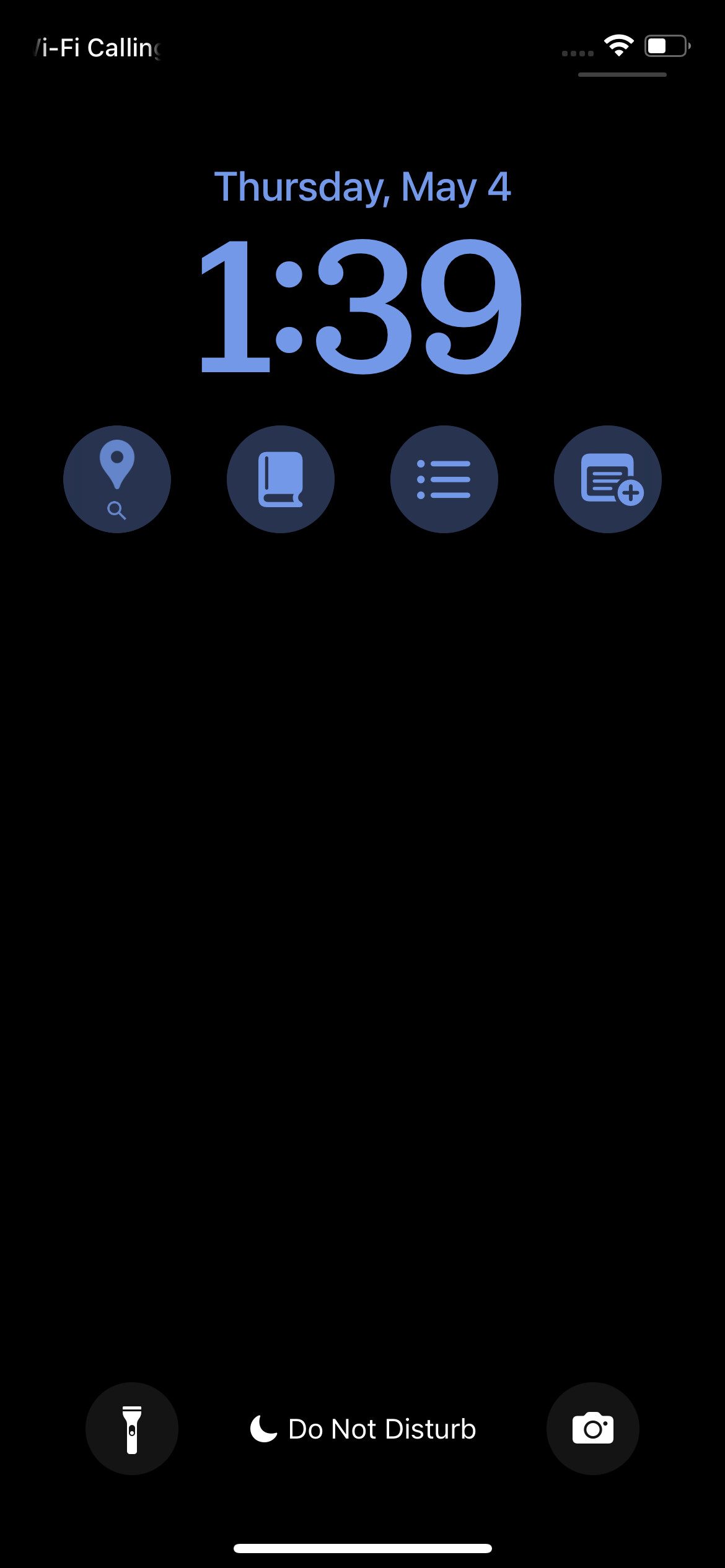This iPhone wallpaper features a sleek, black background. In the top center, it displays the date "Thursday, May 4" in blue text. Below that, the large time display reads "1:39" in a fancy, curly font.

Four circular icons sit prominently below the time, each with a transparent pastel blue background and bright pastel blue symbols. From left to right, these icons depict:
1. A map pin.
2. A magnifying glass.
3. A book.
4. Three dots with corresponding lines.

Situated near the bottom right is a calendar icon with a plus sign enclosed in a circle.

At the very top of the screen, "Wi-Fi Calling" is faintly visible in white text, fading out towards the edges. Alongside this text are four gray dots signifying no service, a white Wi-Fi symbol, and a half-filled gray battery icon with white filling indicating the battery is about half full.

At the bottom left, there is a dark gray circular icon with a white flashlight symbol. The "Do Not Disturb" mode is indicated by a white crescent moon in the middle. On the bottom right, another dark gray circular icon showcases a white camera symbol.

Finally, a bold white line centered at the bottom edge invites the user to swipe up to open the home screen.